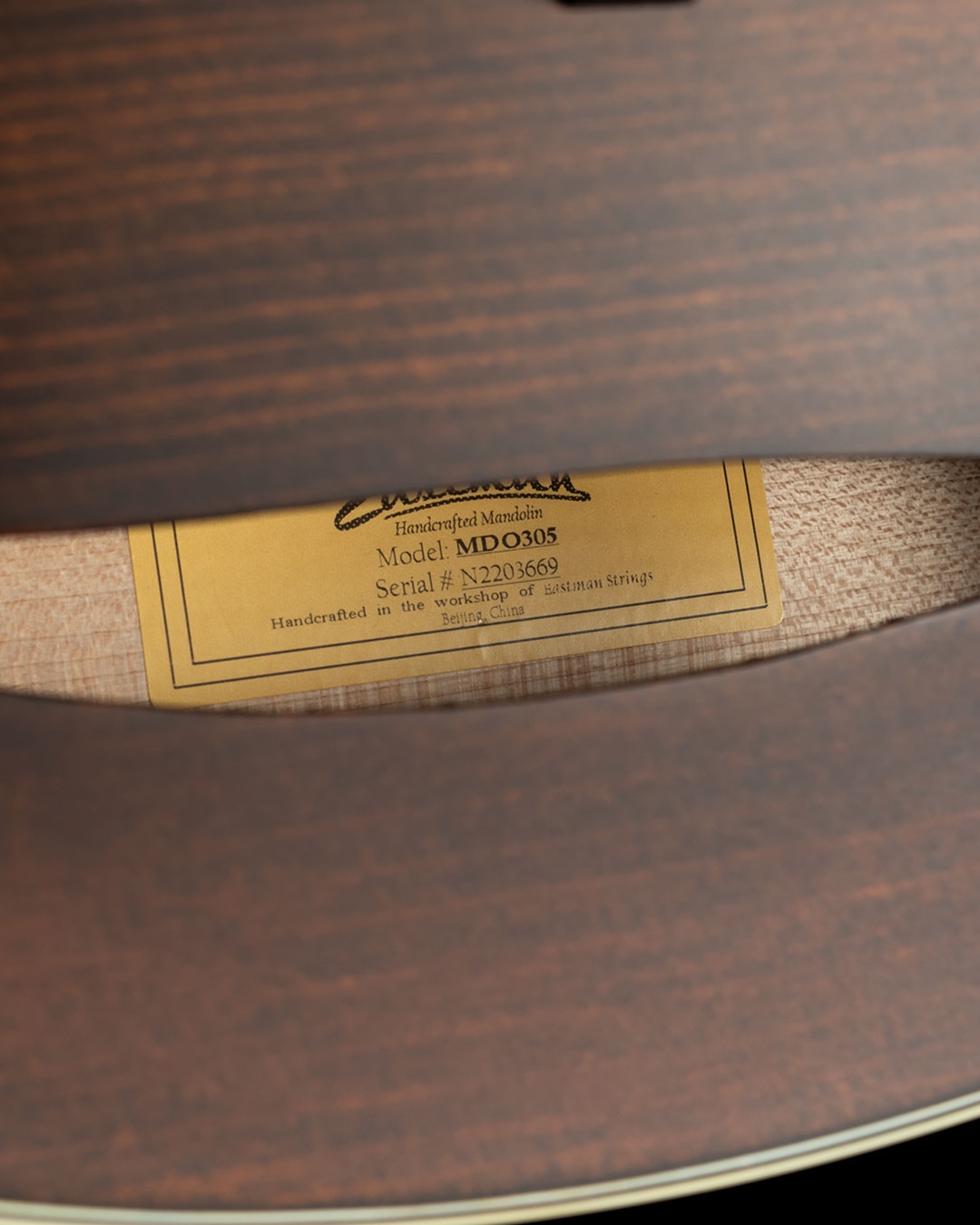The image captures a detailed close-up of a label wrapped around the wooden handle of what appears to be a mandolin. The label is a brassy gold color with black text and lines. Although the brand or product name is obscured by the curvature of the handle, the label features clear text below the logo. It reads: "Handcrafted Mandolin, Model MD0305, Serial Number N2203669, handcrafted in the workshop of Eastman Strings, Beijing, China." The wooden surface of the handle and the surrounding wooden background further suggest that the object in question is indeed a mandolin. The perspective of the shot gives the impression of a magnified view, focusing on the intricacies of the label itself.